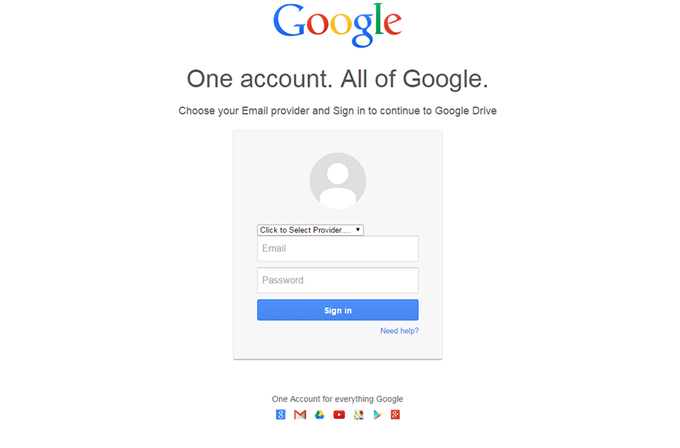The image is a screenshot of the Google login screen with a white background. At the very top, the Google logo is prominently displayed, featuring a blue capital 'G', a red lowercase 'o', a yellow lowercase 'o', a blue lowercase 'g', a green 'l', and a red 'e'. Below the logo, black text states, "One account. All of Google."

Following this, there is a prompt that reads, "Choose your email provider and sign in to continue to Google Drive." Underneath this is a gray rectangle centered on the screen. Within the rectangle, at the top center, there is a circular user icon. Directly below the icon, there is a drop-down menu with the placeholder text, "Click to select provider..."

Beneath the drop-down menu, there are two input fields: the first for the user’s email and the second for the password. Below these fields is a horizontal blue button with the text "Sign In" in white in the center. At the bottom right corner of the gray rectangle, the text "Need help?" appears in blue font.

At the very bottom of the screen, outside the gray rectangle, is a line of text that reads, "One account for everything Google." Following this text are icons for various Google services: the Google logo, Gmail, Google Drive, YouTube, Google Maps, Google Play, and a red square with a 'G' in it.